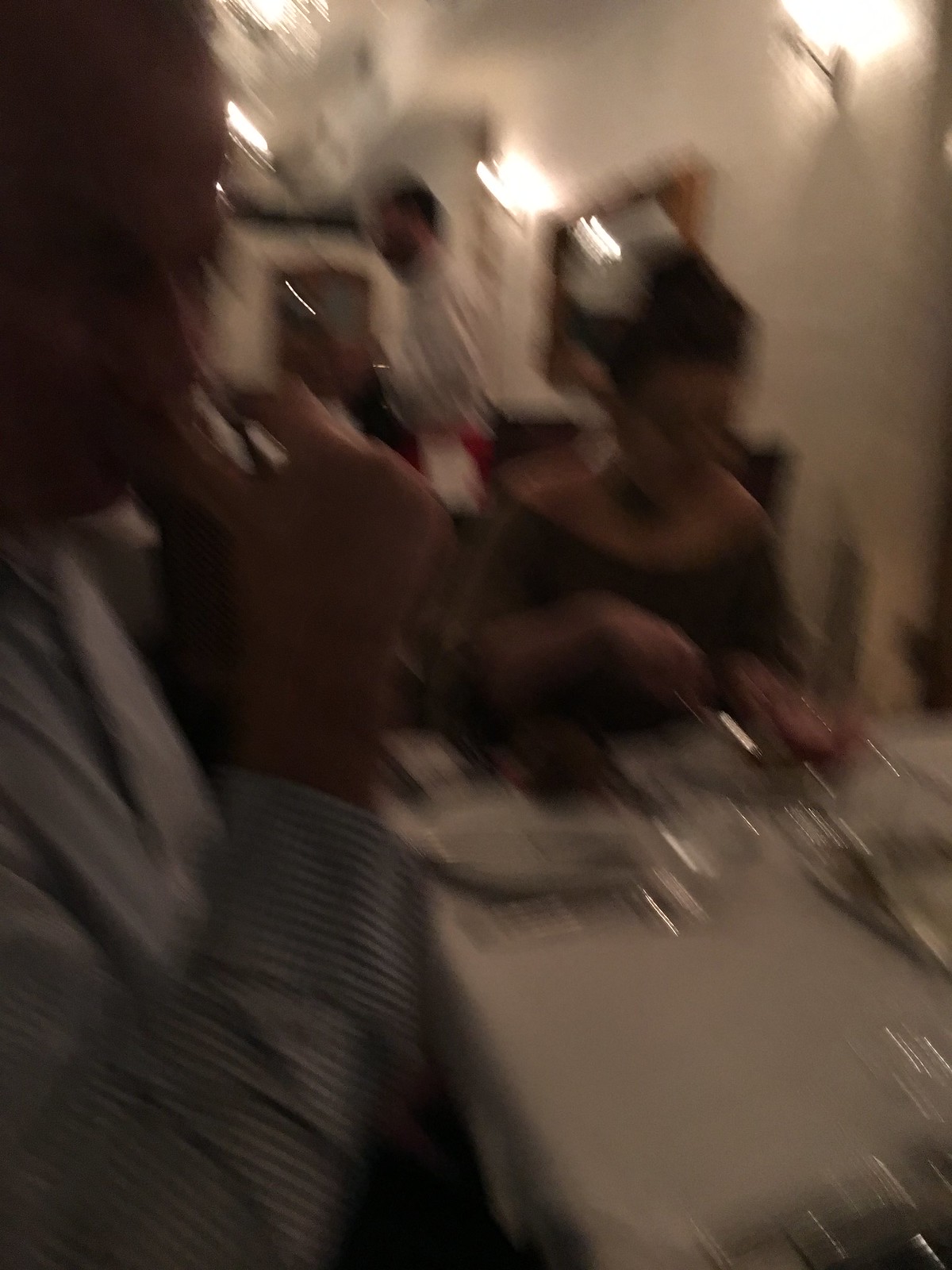This color photograph is significantly blurred and dark, making it challenging to discern specific details. On the left-hand side, a person wearing a dark grey, possibly checkered shirt is partially visible. They seem to be seated at a table set with blurred cutlery and white plates. To their right, a woman with short hair or hair styled up is visible. She is dressed in a dark top with a wide, scooped neckline that appears to be slightly off the shoulder. Behind her, the greyish walls are adorned with a mirror that reflects some light, and blurry light fixtures are mounted on the top. In the background, a person who may be a waiter stands in front of a door, wearing what seems to be an apron around the bottom of their shirt. To the right of the woman, an indistinct white object, possibly another chair, can be seen. There are no other notable elements in the image.